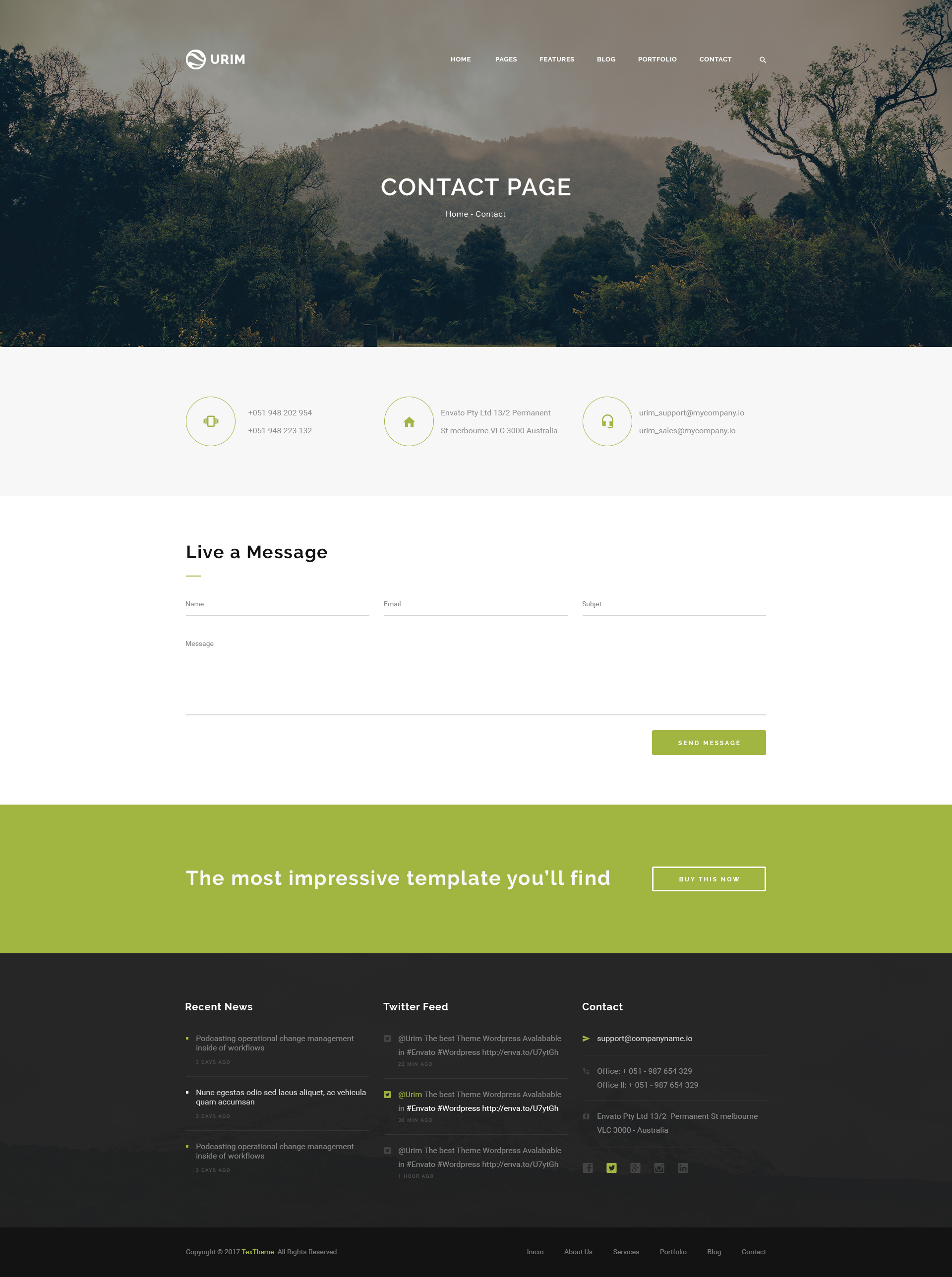**Contact Page of URIM Website**

The contact page of the URIM website features a captivating cover image showcasing a serene mountain nestled within a dense forest. The top navigation bar provides easy access to different sections with links labeled: Home, Pages, Features, Blog, Portfolio, and Contact.

### Contact Information
- **Phone Numbers**: Two numbers are provided, beginning with the international code +051, indicating communication channels in Australia.
- **Company Address**: Envato PTY LTD, 13/2 Permanent Street, Melbourne, VIC 3000, Australia.
- **Emails**:
  - **Support**: support@mycompany.io
  - **Sales**: URIM_sales@mycompany.io

### Contact Form
Visitors are invited to leave a message through the contact form by providing the following details:
- **Name**
- **Email**
- **Subject**
- **Message**

There is a 'Send Message' button for submitting the form.

### Additional Information
At the bottom of the page, there's a tagline promoting the template: "The most impressive template you'll find. Buy this now."

### Footer Section
The footer contains sections with recent news, a Twitter feed, and additional contact details. Each section appears to list three items, although the specific details are not fully visible due to the small font size.

This detailed layout places an emphasis on user engagement and ease of contact, with multiple avenues for visitors to reach out to the company.